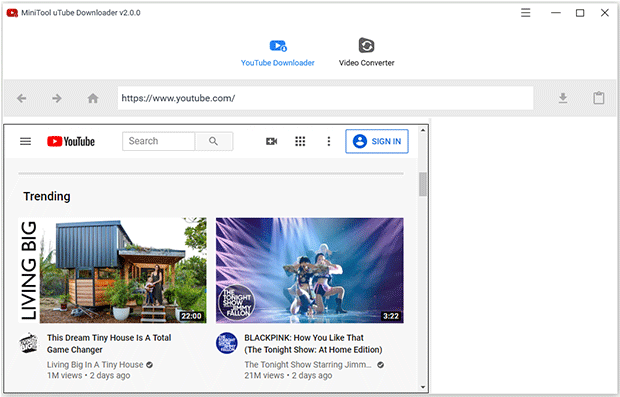The image showcases the interface of MiniTool YouTube Downloader version 2.0.0. At the top, a prominent navigation bar allows users to select between "YouTube Downloader" and "Video Converter" options, with the current focus on the "Downloader" tab. Just below the navigation bar, a YouTube URL has been entered, ready for processing. The interface also features a trending section from YouTube, highlighting popular videos such as "This Dreamy Tiny House is a Total Game Changer" and a performance by Blackpink on "The Tonight Show Starring Jimmy Fallon". The tiny house is depicted as a cozy structure nestled in a woodland setting, while Blackpink is shown performing on a stage bathed in blue light. Additional functionalities of the tool include searching within YouTube, signing in to accounts, and selecting more detailed options for downloading videos. The interface extends further down, though only the aforementioned elements are visible in the image.